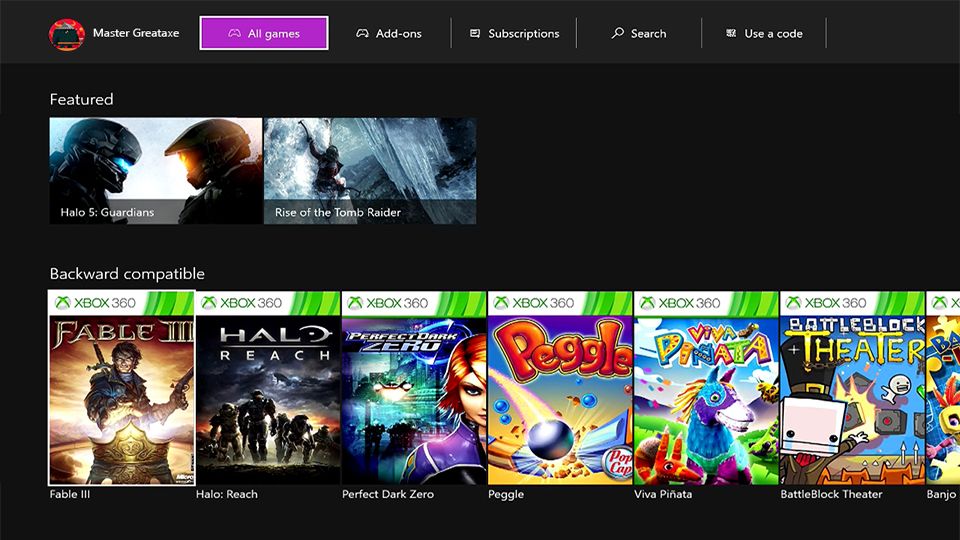The image is a screenshot of a desktop featuring an Xbox account interface. The browser, web address, and operating system are not visible. In the top left corner, there is an icon representing the user named "MasterGreatX." The central focus of the screen is a medium purple rectangle highlighted with a thin white line, showing an icon of a game controller labeled "All Games." 

Other options at the top include icons for "Add-ons" (again showing a game controller), "Subscriptions" (represented by a chat bubble icon), "Search" (indicated by a magnifying glass), and "Use a Code" (with an unclear icon). 

The "Featured" section displays prominent game titles with corresponding images: "Halo 5 Guardians" shows two characters in differently colored helmets facing each other, and "Rise of the Tomb Raider" depicts a character scaling icy terrain. 

Towards the bottom, the category "Backwards Compatible" includes several Xbox 360 titles:
- "Fable 3" shows a figure wielding a sword and gun, seemingly reaching for a crown.
- "Halo Reach" features a cloudy sky and figures, possibly on an alien planet, dressed in mech suits.
- "Project Dark Zero" portrays a woman with short red hair in a purple, possibly futuristic military uniform, set against a cityscape background.
- "Peggle," a game by PopCap, is depicted with elements of a pinball game.
- "Viva Piñata," in bright and colorful font, shows a vividly decorated piñata alongside a small creature resembling a fox or dog.
- "BattleBlock Theater" features a simplistic stick figure leaping and exploding in mid-air, alongside a character with a square face wearing a top hat.

Overall, the screenshot highlights various features, games, and options available to the user on their Xbox account.